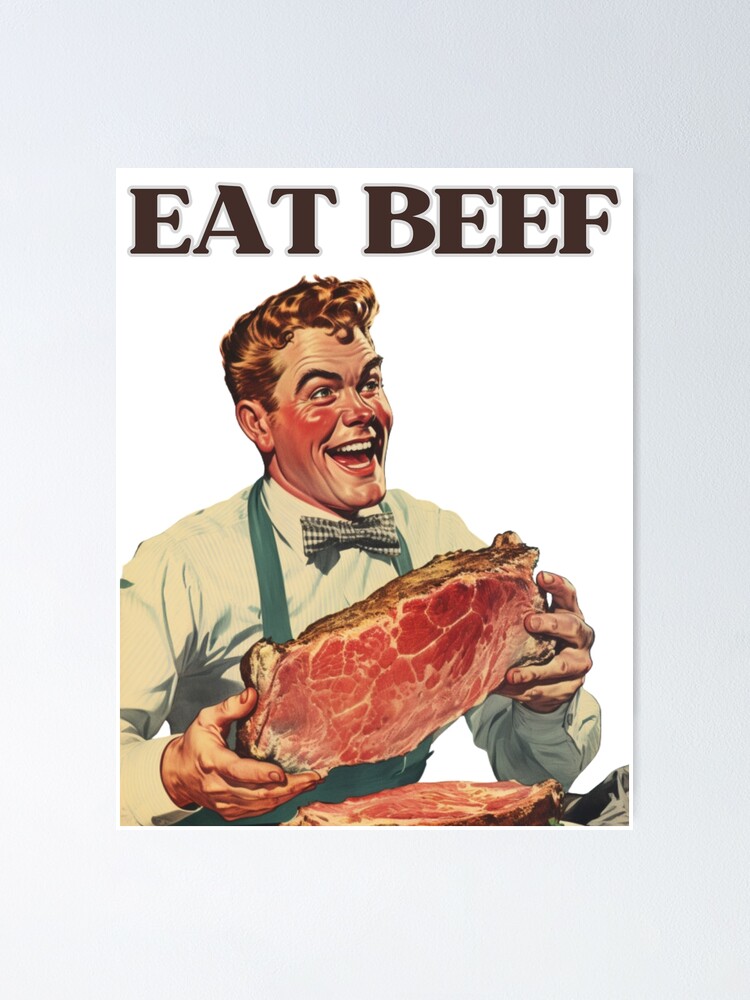This is an artistic illustration reminiscent of 1940s or 1950s cartoon styles, akin to the Saturday Evening Post. Set against a white background framed within a vertically oriented gray rectangle, the illustration features bold black lettering at the top that says "EAT BEEF." Below the text is a cheerful Caucasian man with strawberry blonde hair styled with a little swirl in front and dark black eyebrows. His cheeks are distinctly rosy, and he is grinning widely with his teeth exposed. He is dressed in a white pinstripe button-up shirt with a green polka dot tie (appearing mint green or white), and a green or turquoise apron. The man is holding up a large chunk of beef roast, which appears cooked on the outside but raw with intricate marbling on the inside. His expression is jovial, and he looks off to the right side of the image, adding to the inviting and nostalgic feel of the illustration.